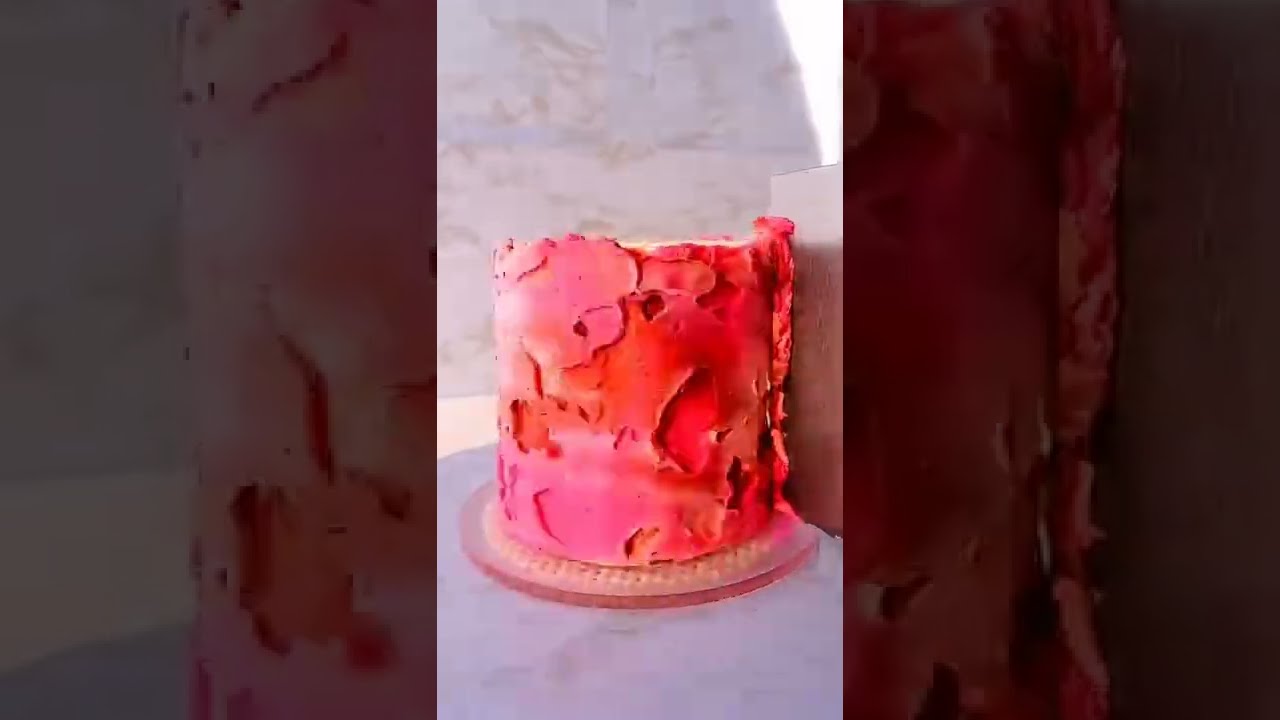The image depicts a circular cake seated on a plate, prominently positioned in the center of a white marble-patterned table. The central third of the image clearly shows the cake, while the left and right thirds display an enlarged and darkened version of the same central photograph. The background features a bright white, grey-veined marble look, suggestive of a kitchen or a bakery environment.

The cake itself is a wide, cylinder-shaped creation enveloped in a textured, abstract icing design. The icing is an eclectic blend of reds, pinks, and occasional hints of orange, with a deliberately uneven, 3D texture. This gives the appearance of a rugged finish, akin to carved stone, rose petals, or candle wax, with some areas exposing a secondary layer of icing beneath. To the right side, a large metal piece, potentially a cake scraper, is poised, suggesting recent or ongoing use to shape the icing. The overall scene is bathed in bright light, possibly indicating mid-day illumination either outdoors or in a well-lit indoor setting.